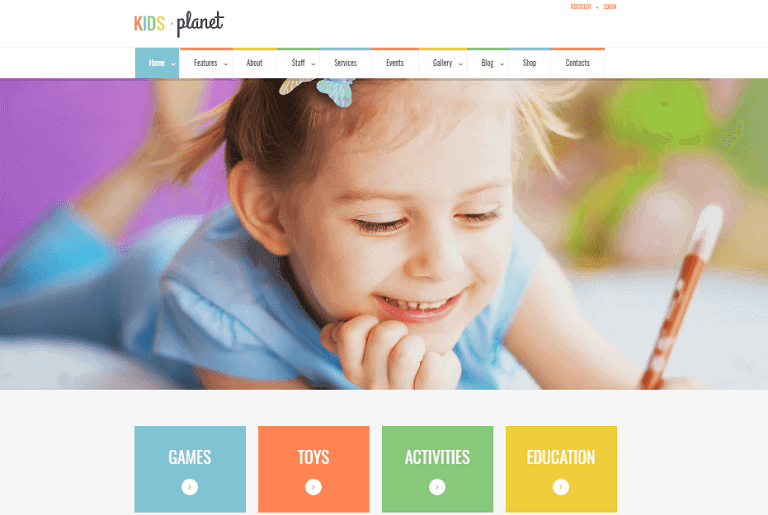This screenshot captures the vibrant and engaging interface of the Kids Planet website. 

In the top left corner, the word "Kids" is presented in a lively multicolored font, followed by "Planet" in elegant black cursive. On the top right, concise orange text denotes the "Register" and "Login" options.

Beneath this header, a navigation bar features sections titled Home, Features, About, Staff, Services, Events, Gallery, Blog, Shop, and Contacts, each labeled in black text against a white background with individual colored tabs for easy identification.

Dominating the page is a large, colorful image of a cheerful little girl engrossed in drawing, her hair tied up with a bow as she smiles brightly, holding a marker.

Below this image are four distinct sections, each vividly colored and labeled in white text: Games on a blue background, Toys on an orange background, Activities on a green background, and Education on a yellow background, offering diverse avenues of engagement for young visitors.